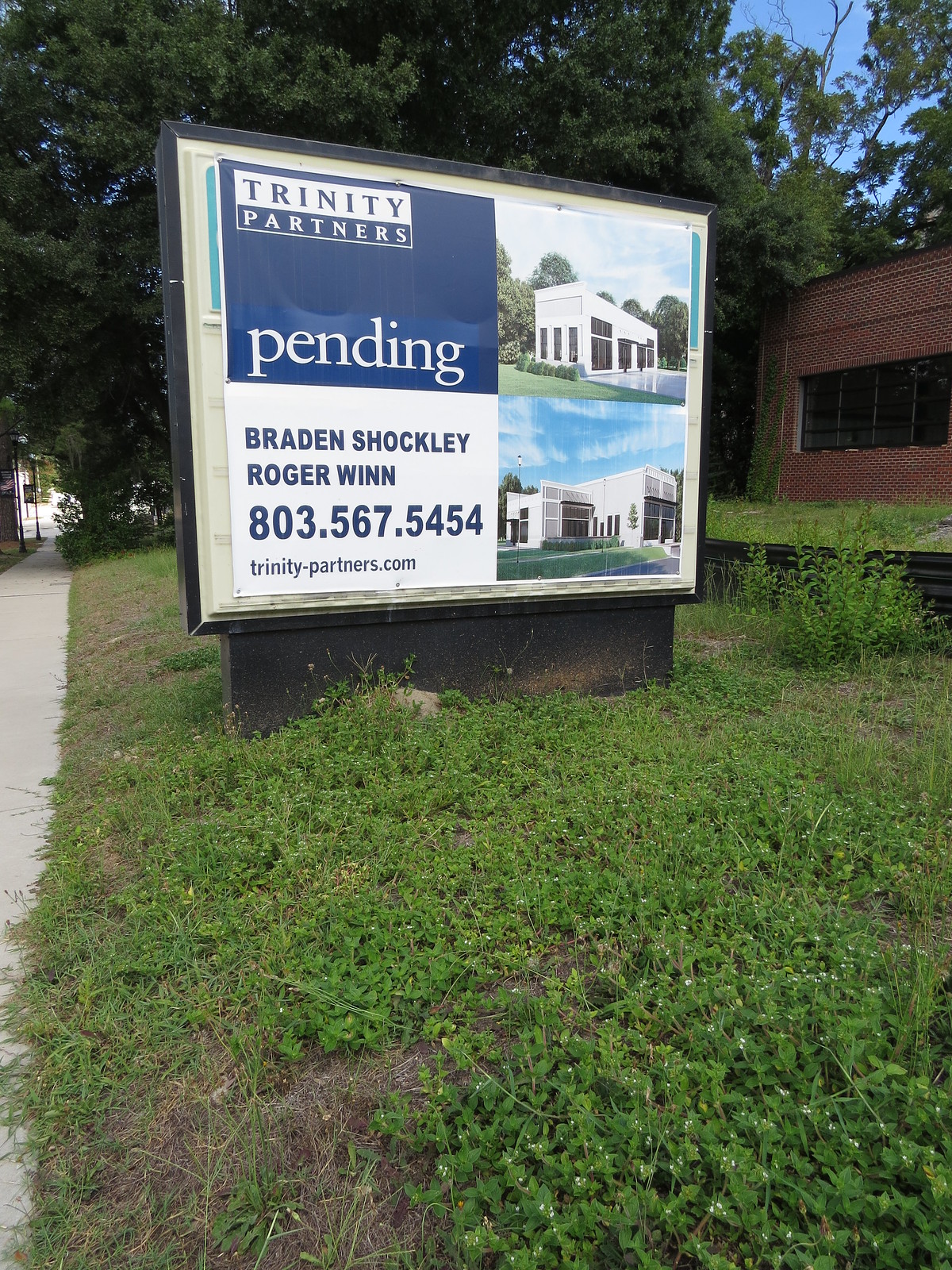The image shows an outdoor scene with a metal sign prominently displaying the name "Trinity Partners" in bold, white text on a blue background, positioned at the top. The sign stands in front of a brick building that appears to be vacant, featuring four large black window panels. Above the building, the sky is clear and mostly blue, with several lush green trees providing a natural canopy. A sidewalk runs along the left side of the image and continues into the background, bordered by overgrown areas with weeds, clover, and grass. The sign also includes a detailed rendering of a proposed white building with arched windows and a pool, labeled with "pending." Below this image, the sign lists names—Braden Shockley and Roger Wynn—in blue text, followed by a contact number, 803-567-5454, and the website trinity-partners.com. This real estate sign clearly reflects the ongoing listing for the development project, captured in a daytime setting.